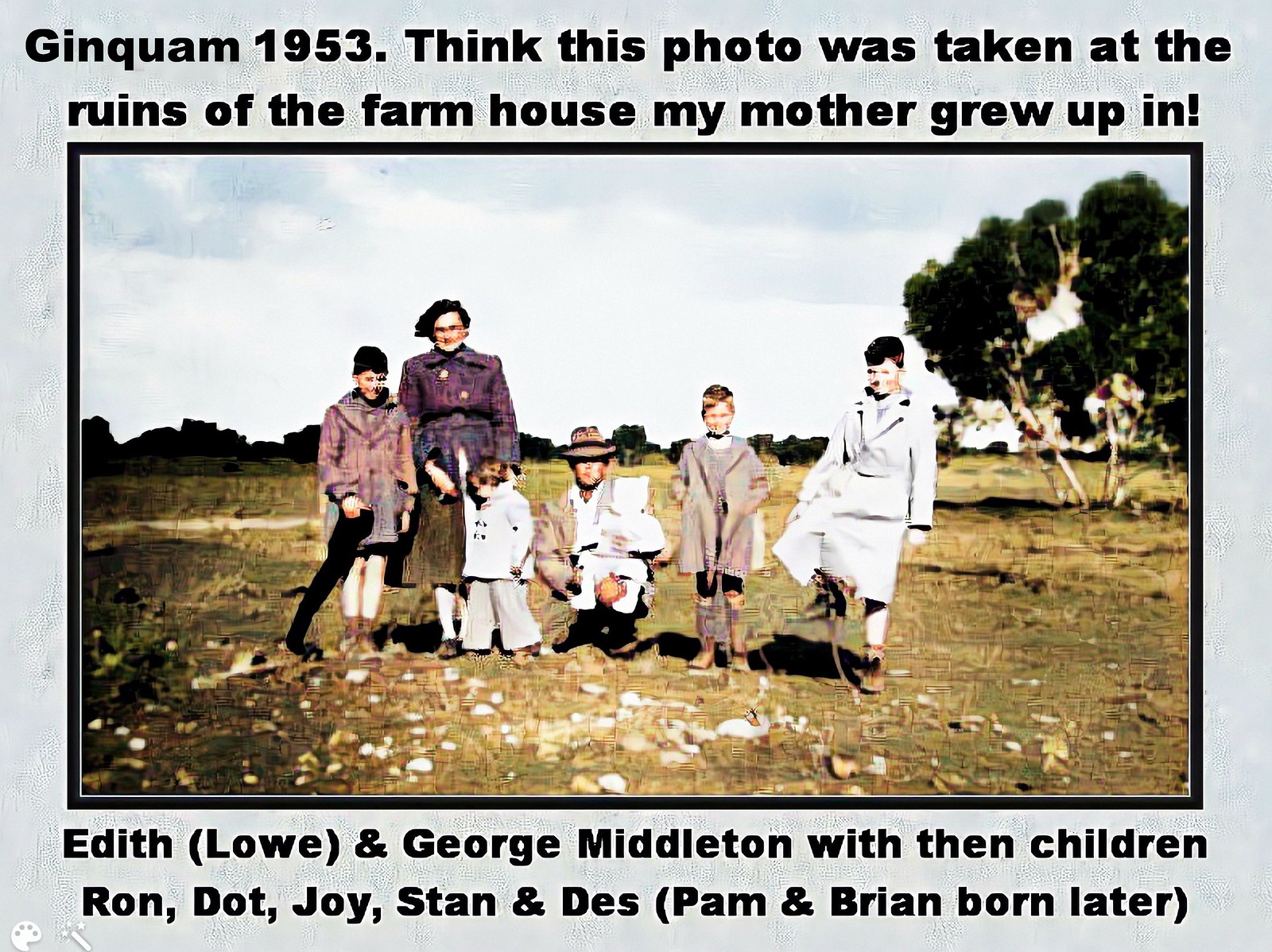The image is a 16x9 horizontal, vintage-style photograph with a color tint added, inset into a slightly larger gray background. The photograph features six individuals standing in a rocky field with trees in the background, facing the viewer. From left to right, there is a dark-haired woman wearing a purple overcoat standing beside two of the four children, followed by a man in the center who is squatting down and wearing a beige top hat. To the right of him are two other young boys, one of whom is balancing on one foot. Black text above the photo reads: "Ginguam, 1953. Think this photo was taken at the ruins of the farmhouse my mother grew up in." Below the image, more text reads: "Edith (Lowe) and George Middleton with their children Ron, Dot, Joy, Stan, and Des. (Pam and Brian born later)." The setting suggests a moment captured during daytime under a lightly clouded sky, adding to the nostalgic and historic atmosphere.